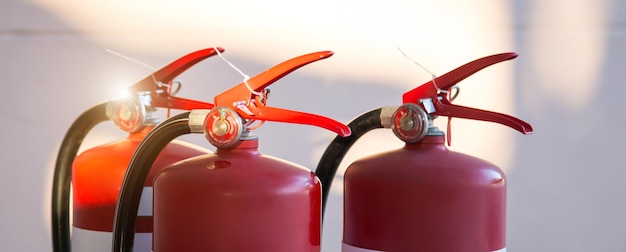The rectangular photograph presents a close-up of the top portions of three red fire extinguishers positioned against a white cinder block wall. The sunlight streams in from the left, illuminating the first extinguisher, which is a bright red with distinct white stripes. This canister is equipped with a bright fiery red handle and a black hose with a steel and rubber nozzle apparatus. Positioned slightly behind the first, the middle extinguisher is a lighter burgundy-red color, features an orange handle, and also carries the functional steel and rubber hose assembly. On the far right, the third extinguisher, characterized by its maroon hue and accented with a white stripe in the middle, includes a red handle. All three fire extinguishers have zip ties around their handles. They are arranged to form a close triangle, with the handles facing to the right and the hoses extending to the left. The overall background alternates between tones of white and gray, with the top portion of the image more brightly lit, emphasizing the sunlit environment.